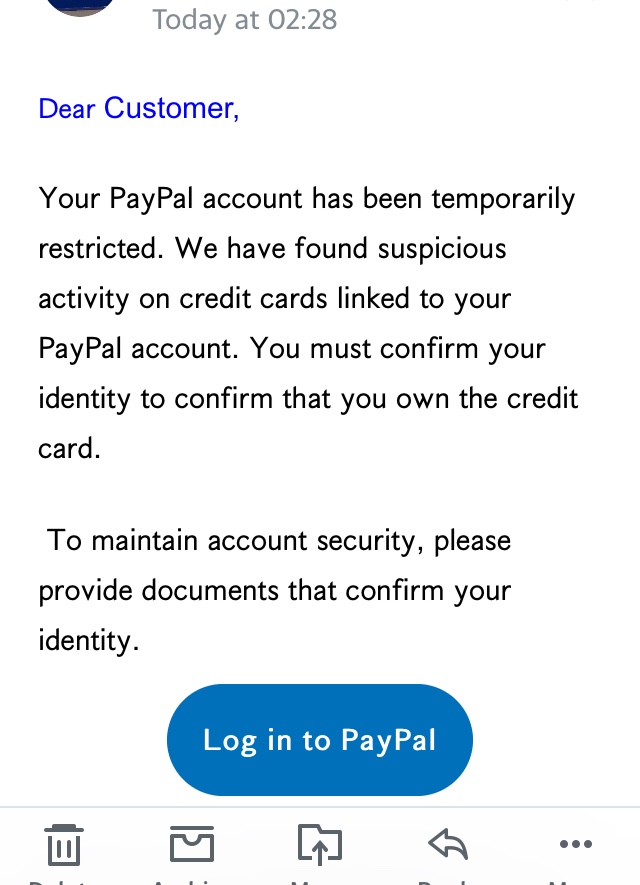This image depicts a screenshot of a section of a website, likely an email interface. At the top of the image, in gray text, it indicates the date and time as "Today at 2:28". Below this, the message begins in blue text with the greeting "Dear Customer." The body of the message is in black text, warning that the recipient's PayPal account has been temporarily restricted due to suspicious activity found on credit cards linked to the account. It requests the recipient to confirm their identity and provide documents to maintain account security. A prominent blue button labeled "Login to PayPal" with white text appears beneath this message.

A gray horizontal line separates the message from a series of icons at the bottom of the screen. The icons depicted are:
- A trash can
- A mailbox
- A folder with an arrow pointing upwards
- An arrow pointing left 
- Three vertical dots

The bottom part of the image is cut off, obscuring the labels for these icons. Similarly, the top part of the image is truncated, cutting off most of what appears to be a profile picture, leaving only the bottom curve of a circle visible.